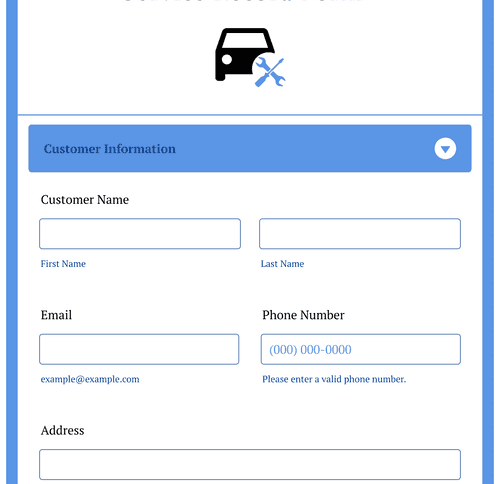This website form is visually structured with distinct sections and clear color coordinates for user navigation. The layout features a blue strip running vertically along both the left and right sides. The top visible section is predominantly black with a white circle positioned to the left. 

Centering the form, the windshield appears trapezoidal and white. Adjacent to the 'Wheelie Pool' on the right, another white circle is visible. Below are two tool icons, one colored in blue, potentially representing either a screwdriver or a wrench.

Below this initial band, a prominent white line horizontally divides the page. It includes a blue rectangle on the left side, shaded in a darker blue which says 'Customer Information'. Opposite on the right, another white circle hosts a blue downward-pointing triangle.

The background transitions to white for the form's fields. The text 'Customer Name' is printed in black on this backdrop, preceding two adjacent rectangles bordered in blue. On the left rectangle's upper-left corner, there’s the label 'First Name' in blue. Similarly, the right rectangle’s label, 'Last Name', appears with adequate spacing for user input.

Proceeding this section, similar pairs of boxes appear for 'Email' and 'Phone Number'. The 'Email' field is pre-filled in black with 'example@example.com' as an illustrative placeholder. For 'Phone Number', a note in blue encourages users to enter a valid number, represented in parentheses as (000-000-0000).

The meticulous design employs a crisp contrast of colors ensuring clarity and ease of use.